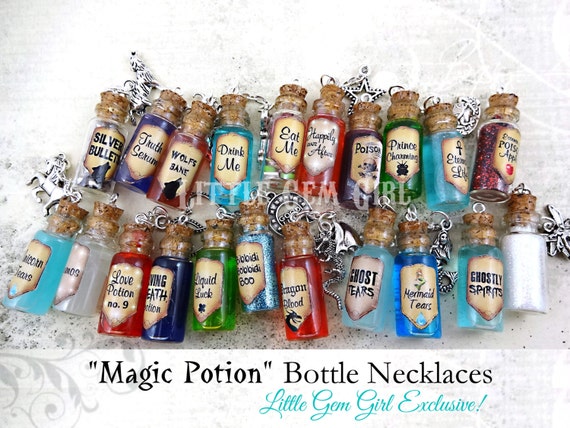This is an artistic photo showcasing an array of approximately 20 small, vintage-style glass bottles, each sealed with a cork and filled with various colorful liquids. The bottles, varying hues from aqua blue, vivid dark blue, red, pink, green, purple, clear, and even glitter-filled, are meticulously arranged on a textured, grey and white backdrop. These bottles have charming, old-timey brown labels that evoke a Renaissance feel, inscribed with enchanting names such as "Ghost Tears," "Drink Me," "Silver Bullet," "Prince Charming," "Ghostly Spirits," "Liquid Luck," "Love Potion," "Truth Serum," "Wolfsbane," "Happily Ever After," "Poison," "Mermaid Tears," and "Bibbidi-Bobbidi-Boo," among others. Some of these bottles are attached to chains, making them wearable as whimsical necklaces. Underneath the display, in black and white lettering, is the phrase "Magic Potion Bottle Necklaces by Little Gem Girl Exclusive!" capturing the magical essence of these ornamental accessories.